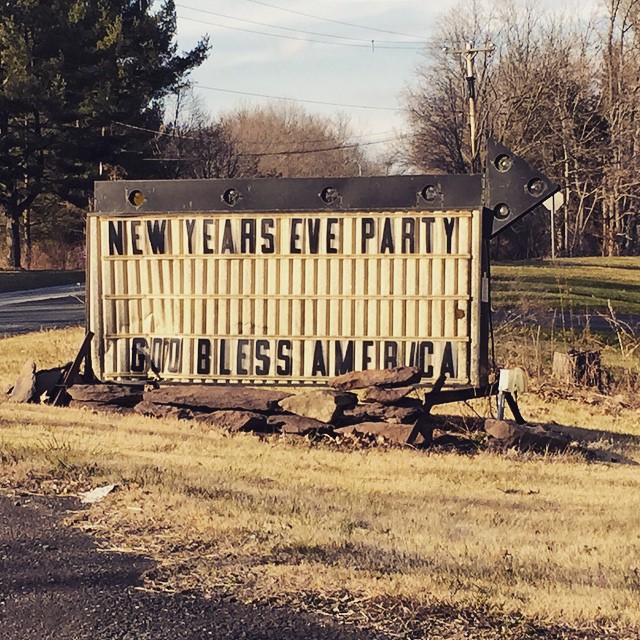This photograph captures a roadside sign set against a vivid backdrop of the blue sky with white clouds. The sign sits prominently in the center, bearing the message "New Year's Eve Party" at the top and "God Bless America" at the bottom, both in black text on a white paneled background. A large black arrow, extending off to the right, crowns the sign. This arrow features cutout areas with four bolts running down its length and three more within the arrow itself, designed to light up.

The sign is supported by angled brackets and surrounded by a pile of brown rocks or shale, resting in a light brown, sun-worn grassy area. To the left of the sign lies a foreground patch of black gravel. The setting appears to be a roadside location with an asphalt road nearby.

In the background, there are numerous trees, including a prominent green tree on the top left and several leafless trees further to the right. Scattered throughout are electrical poles with lines extending in various directions, adding an element of rusticity to the scene.